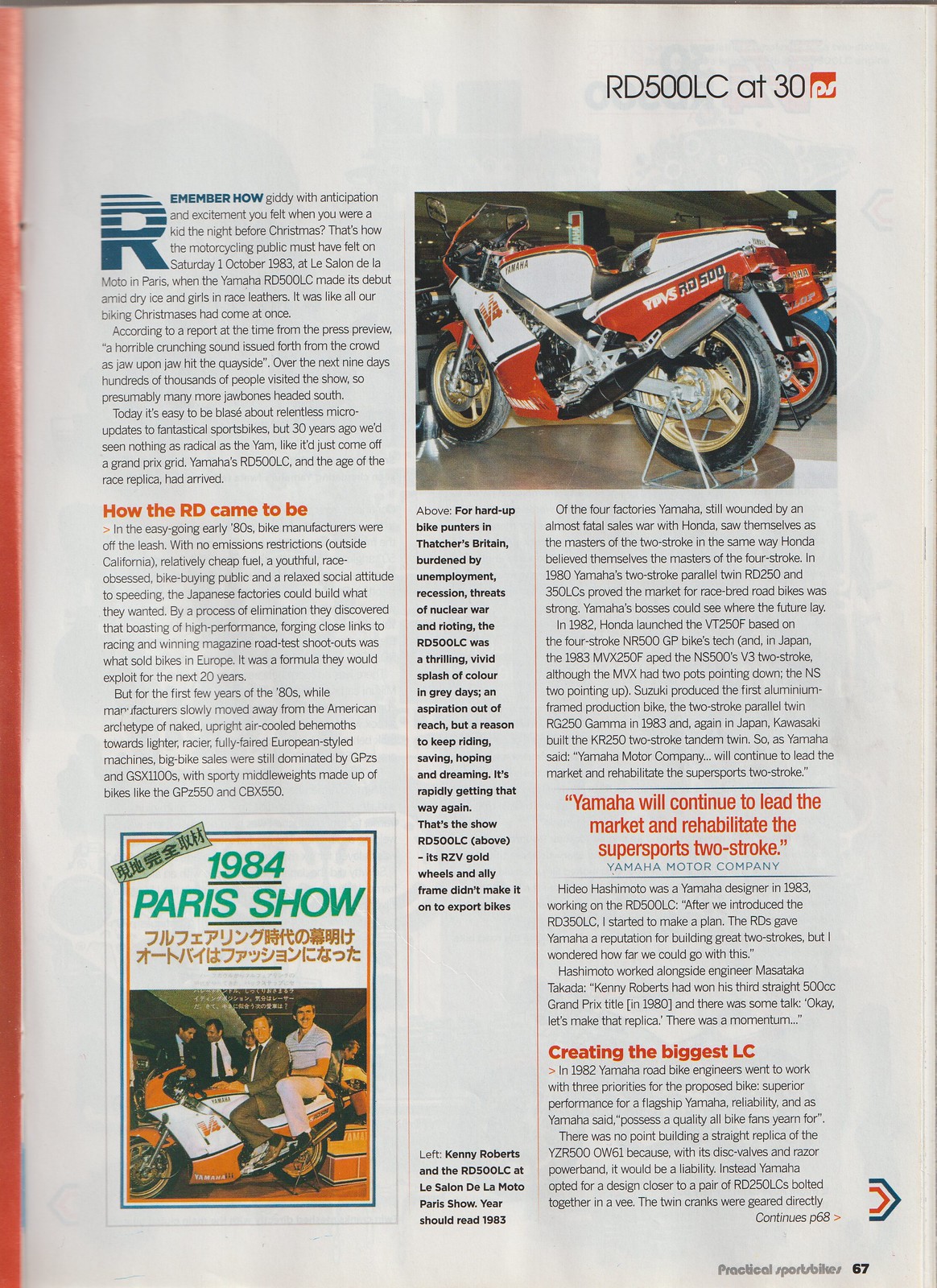This magazine page, marked as page 67, features content about motorcycles, primarily focusing on the 1984 Paris Show. The top left corner showcases a large teal 'R' followed by the phrase "Remember How?", with the text below discussing the history and market influence of Yamaha's RD series. The article includes details about Yamaha's strategy to continue leading the market and revitalizing the Supersport 2-stroke category while creating the biggest LC.

On the right-hand side, there's a prominent photograph of a red, white, and black motorcycle facing left, drawing attention with its sleek design. Toward the bottom right corner, there's another image depicting several men with motorcycles. One man sits on a red and white motorcycle, similar to the one shown above, with another man behind him and additional men in the background. A caption below this image states "1984 Paris Show," along with text in Japanese or Chinese. The page is densely packed with text in various languages, including small black prints and some larger, easier-to-read phrases in red. Notably, key phrases like "how the RD came to be" and "Yamaha will continue to lead the market and rehabilitate the Supersport 2-stroke" are prominently displayed. The left edge of the page features a vertical orange strip, adding a visual break to the layout.